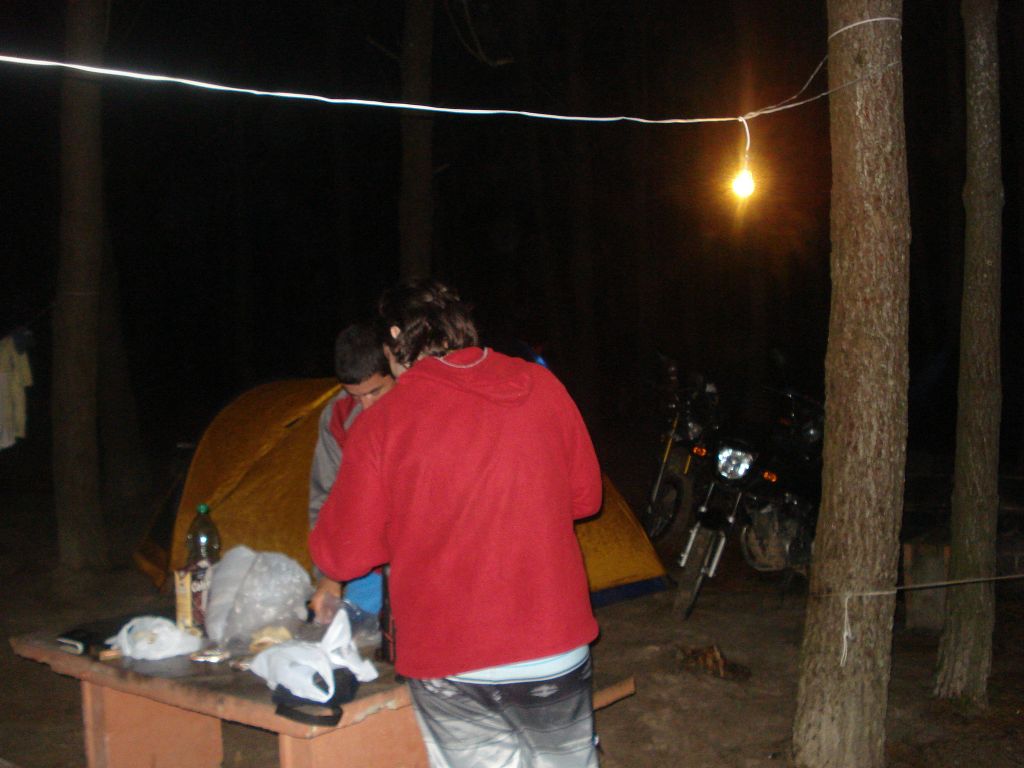The photograph captures an outdoor nighttime scene at a campground. The image prominently features two men near a table cluttered with items including white plastic bags and a green bottle. The man in the foreground is wearing a red shirt, has his back to the camera, and is dressed in black pants that hang low, revealing the band of his underwear. To his right, a motorcycle is parked, reflecting the camera's flash off its headlight. Above him, a single light bulb hangs from a wire, casting a dim glow. Behind him, partially obscured, is another man wearing a gray jacket and looking down. A pair of tree trunks with a rope or string between them stands to the right of the scene. The background reveals glimpses of an orange dome tent among the trees. The setting suggests that the group is camping, with the motorcycles and tent enhancing the atmosphere of a casual, nighttime gathering.